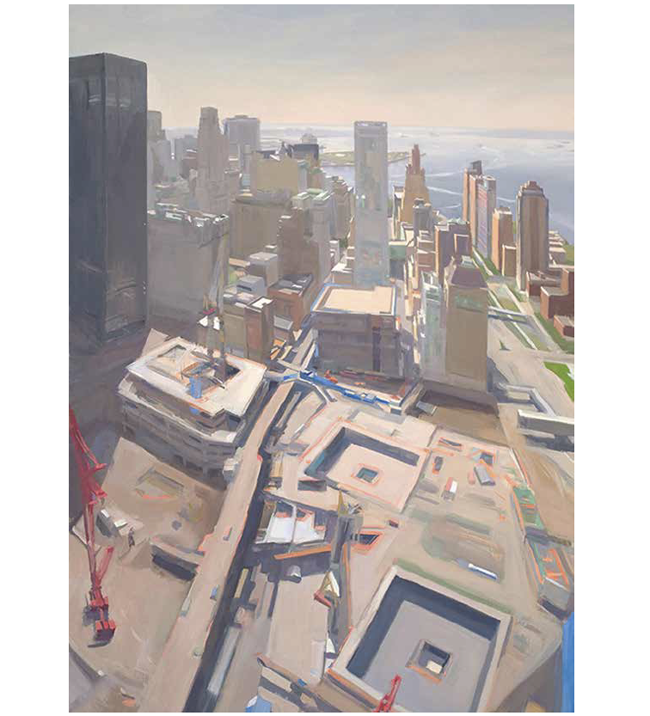This is an overhead wide-angle shot of a high-rise building under construction, depicted as an art piece painting. The top of the building features three large, square holes where additional structural supports are being built. Dominating the lower left corner is a large red crane, near which stands a person directing the construction activities. Adjacent to the crane, on the left side, is a portion of the building characterized by a sleek, black glass tower accentuated with reflective surfaces. The top left corner also reveals an antenna contributing to the intricate skyline. Surrounding the construction site are other high-rise buildings, forming a dense cityscape that extends toward a waterfront visible in the upper right corner. The background reveals the expanse of blue-gray ocean waters meeting a softly colored sky, blending seamlessly with the light, neutral tones of the entire composition. The painting captures both the dynamic urban development and the serene natural elements coexisting within the city's architectural framework.